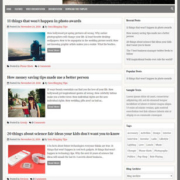This image is a very blurry screenshot of a web page, making it difficult to read the details. The background on both sides is a dark gray, with two vertical stripes. The layout suggests that it is a web app, featuring three rows each containing what appears to be a thumbnail image. There aren’t any visible prices, indicating it might be related to movies rather than a shopping site.

At the upper center of the image, there is a noticeable black stripe with a faint light source at the far right. Below this is another dark gray stripe, obscured to the point where text is illegible. This stripe appears to contain five tabs.

Beneath the tabs are three rectangular sections of information. Each section has an image located at the bottom left corner. The red description text is also present but blurred. From what can be discerned, the middle rectangle seems to depict two girls hitchhiking. The top rectangle might show a building, while the bottom rectangle has what looks like a pad of paper and a watch against a black background.